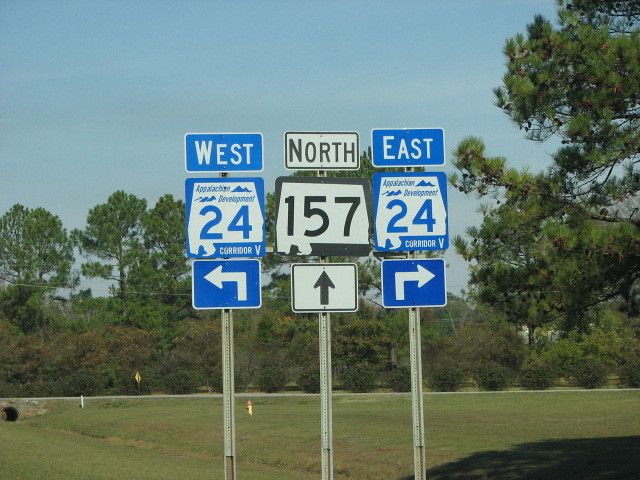This is a rectangular photograph, taken as if from a moving vehicle, which captures three freeway signs aligned in a row. The left sign, blue and white, is topped with the word "West" in white letters against a blue background, followed by "Appalachian Development 24 Corridor V" in a bluish-white field, and a white-outlined blue arrow pointing left. The middle sign features a black and white palette, stating "North 157" above a straight arrow. The rightmost sign mirrors the left in style, displaying "East 24 Corridor V" and a right-pointing arrow. The signs are mounted on three metal poles and set against a verdant backdrop—a vast green field stretches towards tall trees, accompanied by lower shrubbery and brush. Notable details in the scenery include a bright green tree adorned with pine cones, which casts a shadow to the left, a fire hydrant in the middle of the field, and a drainage system towards the far left. Above, the sky is a clear, uninterrupted blue.